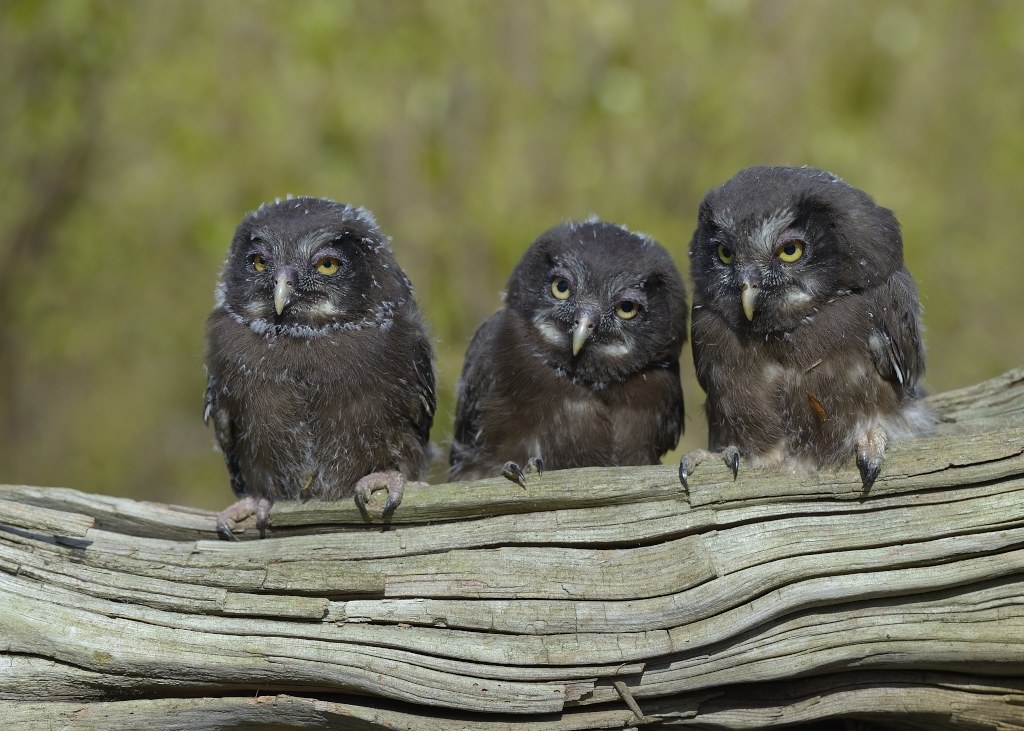This image features three juvenile owls perched closely together on a weathered, grayish-white log with numerous splits and parallel cuts. Each owl, covered in dark brown and black downy feathers, grasps the log with their curved claws. Their vibrant yellow eyes with black pupils are wide open, giving them a curious, attentive look. The owl in the center appears slightly shorter, leaning to the right, while the other two gaze directly at the camera. The blurred background hints at a natural setting with various shades of green and indistinct trees. The overall scene is well-lit, suggesting it was taken outdoors, possibly in a professional or portrait mode setting.